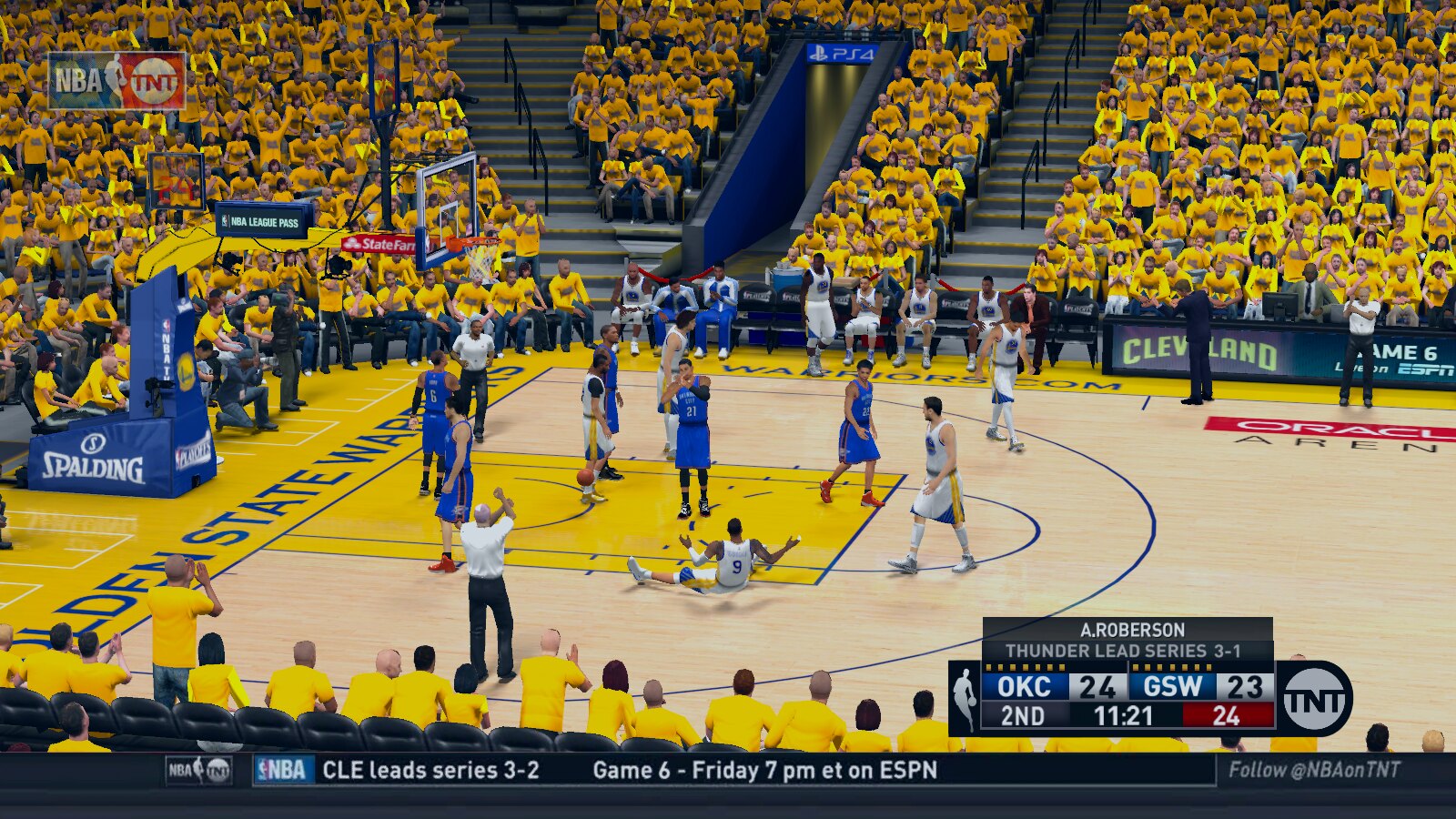A screenshot from an NBA-themed PlayStation 4 video game. The top left corner displays the NBA and TNT logos. Along the bottom, an informative ticker reads: "CLE lead series 3-2 Game 6 Friday 7 p.m. on ESPN" followed by "Follow @NBA on TNT." Additionally, a rectangular box indicates the score and game specifics: "Robertson Thunder lead series 3-1, OKC 24 - GSW 23," with 11:21 remaining in the second period. The Golden State Warriors' home court is evident, complemented by animated fans wearing yellow, characteristic of the digital in-game environment.